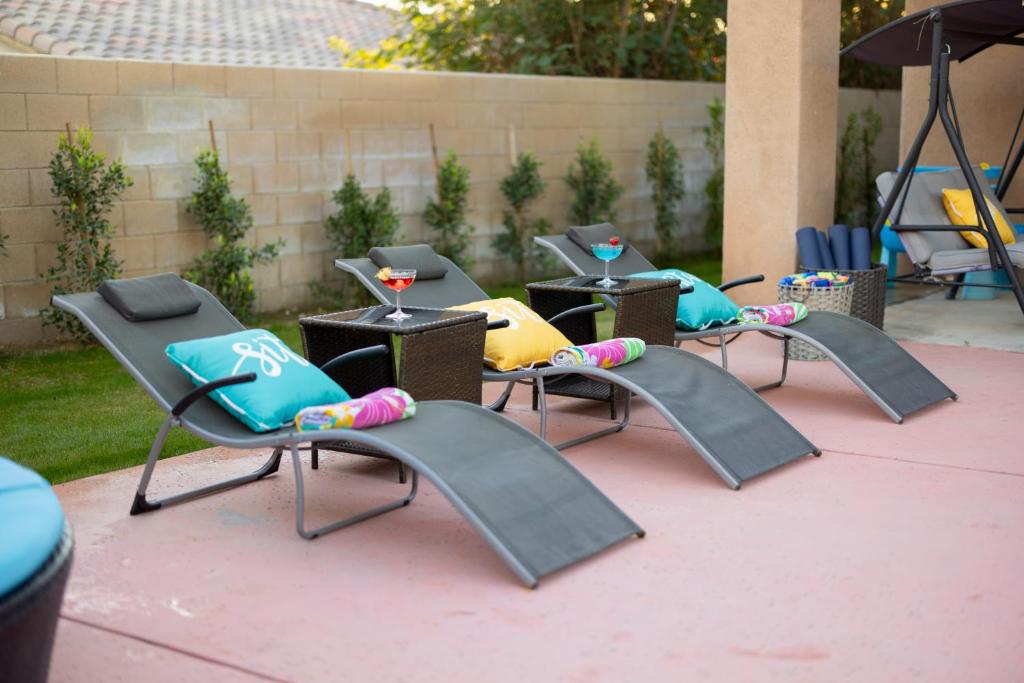This horizontal color photograph captures an inviting outdoor poolside scene, likely at the back of a home or hotel, though the pool itself is not visible. The focus is on three black mesh chaise lounges, each equipped with a colorful pillow—two turquoise and one yellow—and a neatly folded towel. Between each lounge sits an outdoor wicker table with a glass top, each holding a vibrant, beachy cocktail. The setting suggests preparation for guests, with additional baskets off to the right containing more beach towels and pool noodles. The scene is framed by a well-kept green lawn and an 8-foot tall cinder block fence with young plants staked for growth, hinting at future blooms. The pink concrete patio underpins this serene arrangement, adding a subtle warmth to the scene, completed by the partial glimpse of a swinging chair to the right.